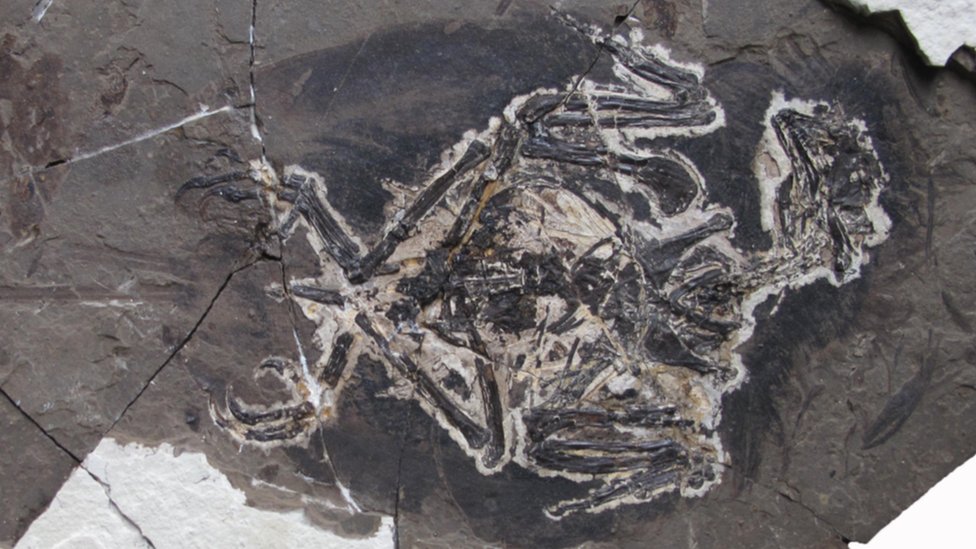The image depicts a section of what appears to be a stone or pavement ground, seen from a direct overhead perspective. The surface is cracked and features a design that vaguely resembles the skeletal remains of a bird, suggesting an intricate pattern etched into the stone. The stone itself has varying shades of white, black, and gray, with a wet appearance, particularly noticeable in the lower left-hand corner where a white chunk of rock lies amidst the darker, moistened surface. This design, positioned more towards the center right of the image, is somewhat enigmatic and could either be an artistic engraving or a natural formation resembling a petrified bird. The bird-like pattern shows distinctive features such as wings, legs, a head with a beak, and what seem to be preserved feather-like details surrounding it, lending a sense of an archaeological find. The absence of text or additional objects in the image leaves its exact nature open to interpretation, but the detailed cracks and the evident drying liquid add depth to the intriguing setting.